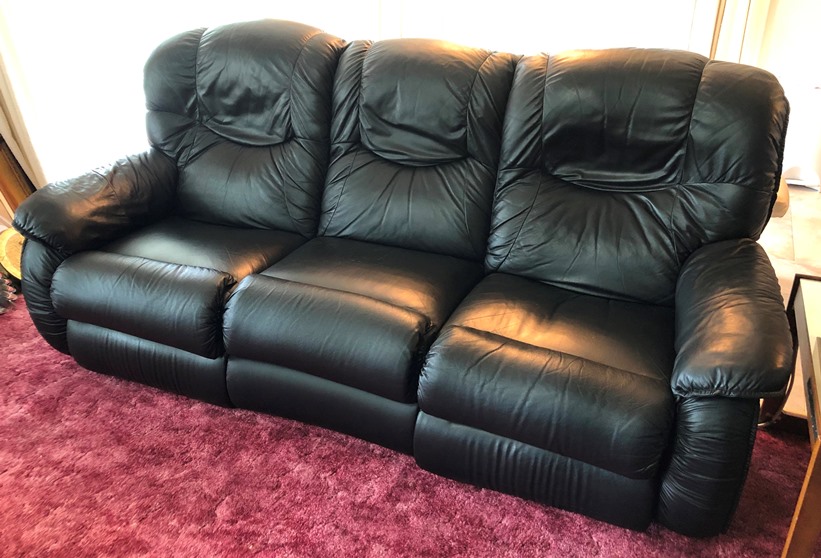The photograph features a luxurious, three-seater black leather couch, prominently situated on a plush, shaggy carpet that shifts in color between a rich rose pink and subtle purple, adding a cozy ambiance. This puffy and soft couch is divided into three distinct sections, each with well-padded headrests and cushy armrests on either side, emphasizing its comfort and inviting appeal. The lighting in the room creates an interesting visual effect; a bright, possibly overexposed, white light spills from what appears to be a window behind the couch, casting a gentle golden sheen on parts of the seats. Additionally, a partial view of an end table with orange legs and a whitish, translucent tabletop is visible on the left side of the couch, while a white table with squared wooden legs is noted on the right side of the image. The overall scene is slightly tilted to the right, contributing to a dynamic yet homely aesthetic.